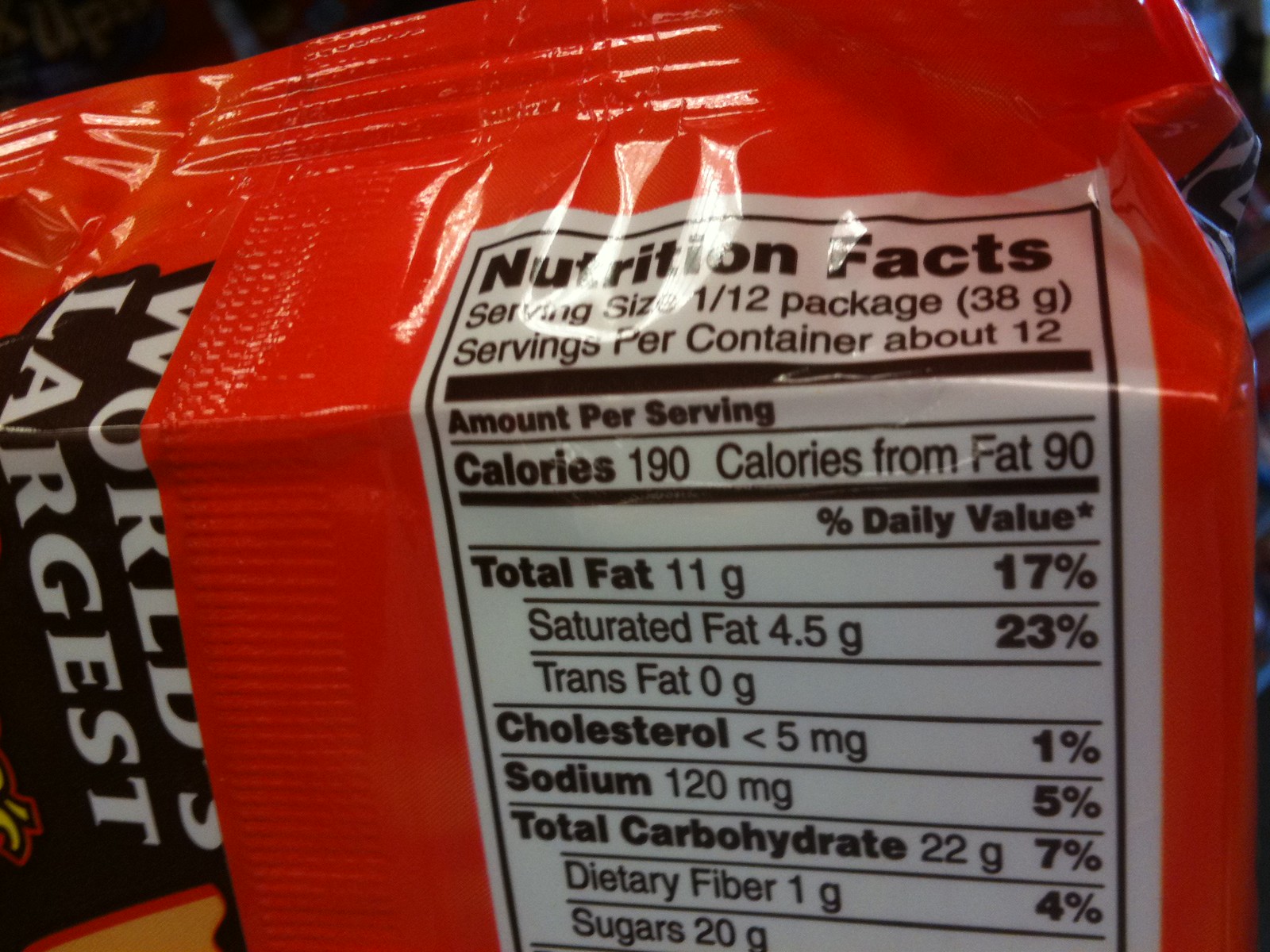This first-person POV close-up photograph depicts the back of a glossy, red plastic snack bag, which is likely a chip or crisp package. The package has a structured, possibly box-like form. Prominently featured on the left side, turned vertically, are the words "World's Largest" in white bold text on a black background. Alongside the right side of the pull tab, the detailed Nutrition Facts are displayed against a white box in black text. Key nutritional information includes a serving size of 38 grams (1/12th of the package), 190 calories per serving, with 11 grams of total fat (17% daily value), 4.5 grams of saturated fat (23% daily value), 0 grams of trans fat, less than 5 milligrams of cholesterol (1% daily value), 120 milligrams of sodium (5% daily value), 22 grams of total carbohydrates (7% daily value), 1 gram of dietary fiber (4% daily value), and 20 grams of sugars. A hint of a yellow graphic peeks out from the bottom left corner of the image.